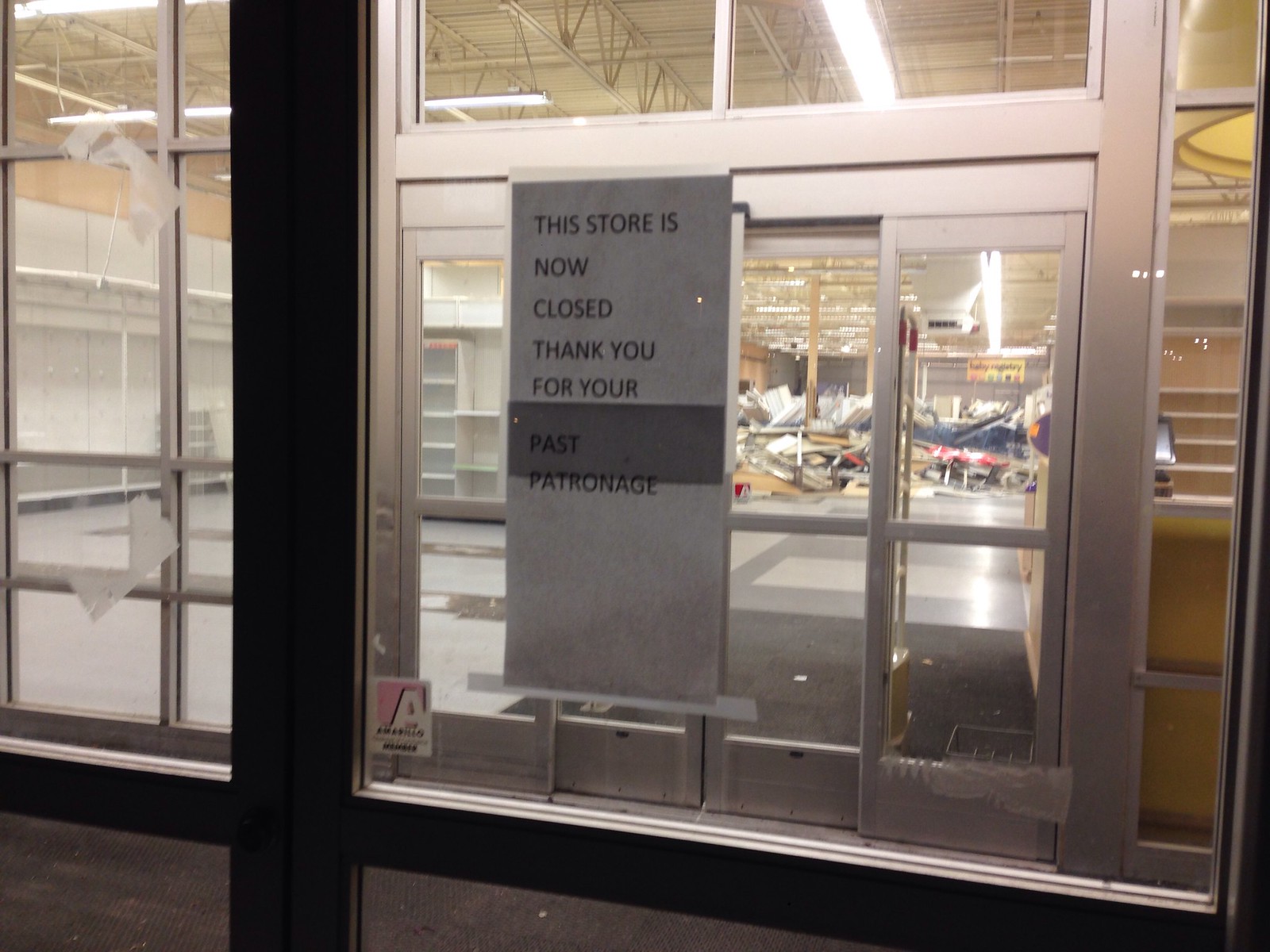This photo captures the entrance of a store with a disheartening scene inside. The entrance features two successive sets of sliding glass doors; the first set has a black trim, followed by a second set with a white trim. Through these doors, you can glimpse into the interior of the store where the shelves, once laden with goods, now stand empty. In the far background, the store appears to be in disarray, with debris and various items chaotically piled on top of one another, suggesting some form of extensive destruction. A sign on the front door poignantly announces that the store is now closed, expressing gratitude for past patronage. Despite the mess, a countertop on the right side remains intact, still holding a computer, hinting at the normalcy that once was.